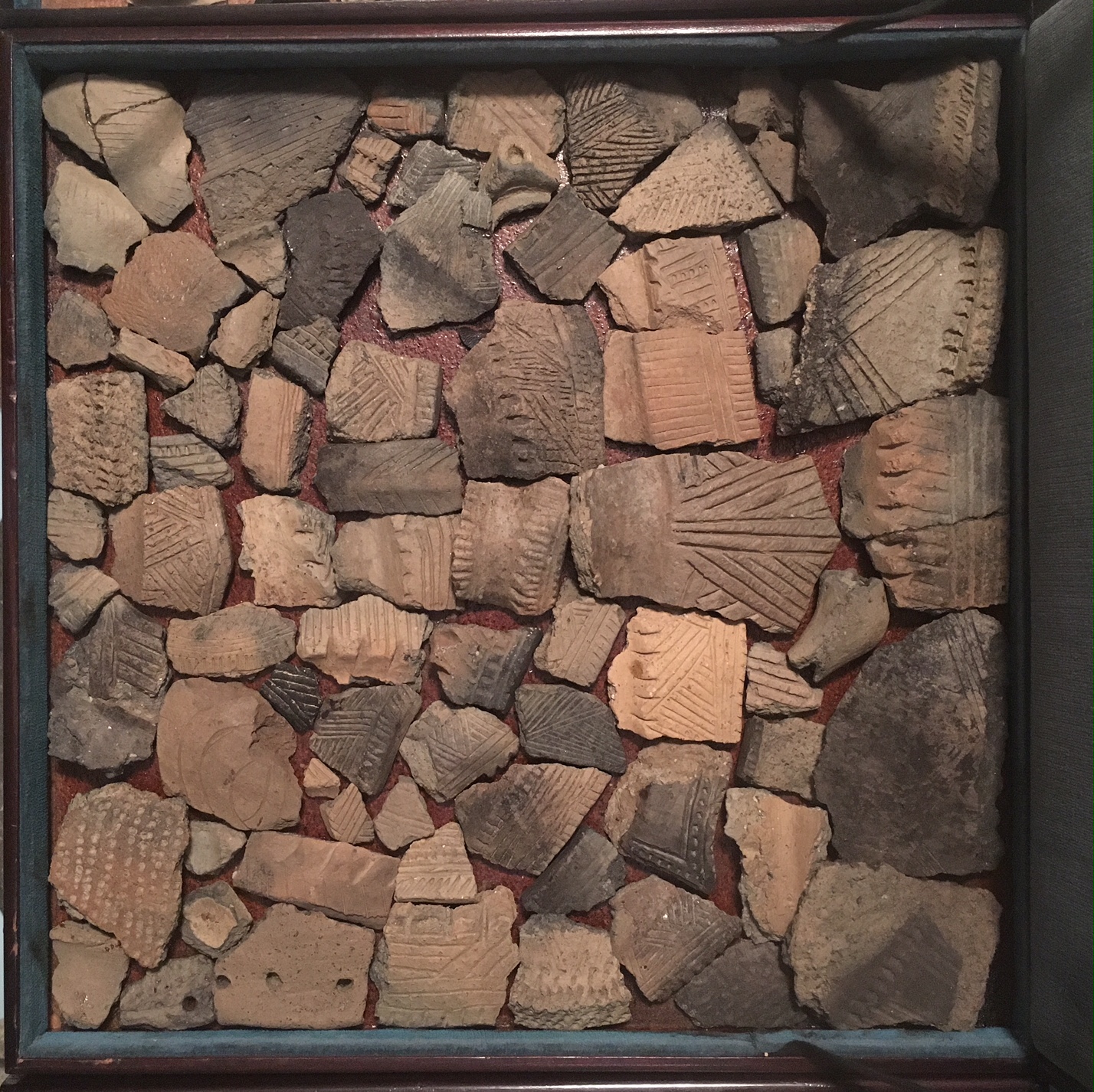The image depicts a meticulously arranged display of ancient artifacts, likely broken ceramics or pottery, set against a richly maroon-colored background. The fragments vary in size and shape, with some distinctly slanted and cracked, creating an impression of disjointed yet deliberate assembly. Encased within a dark, possibly wooden frame, these pieces are organized in a collage-like manner. Noteworthy fragments include a brown piece with vertical and diagonal lines, smaller black shards, a red piece adorned with white dots, and a light tan fragment featuring black stripes. The dark frame accentuates the different colored ceramics, while the arrangement suggests a careful excavation and preservation effort, with some pieces appearing to have been reassembled from their broken states.